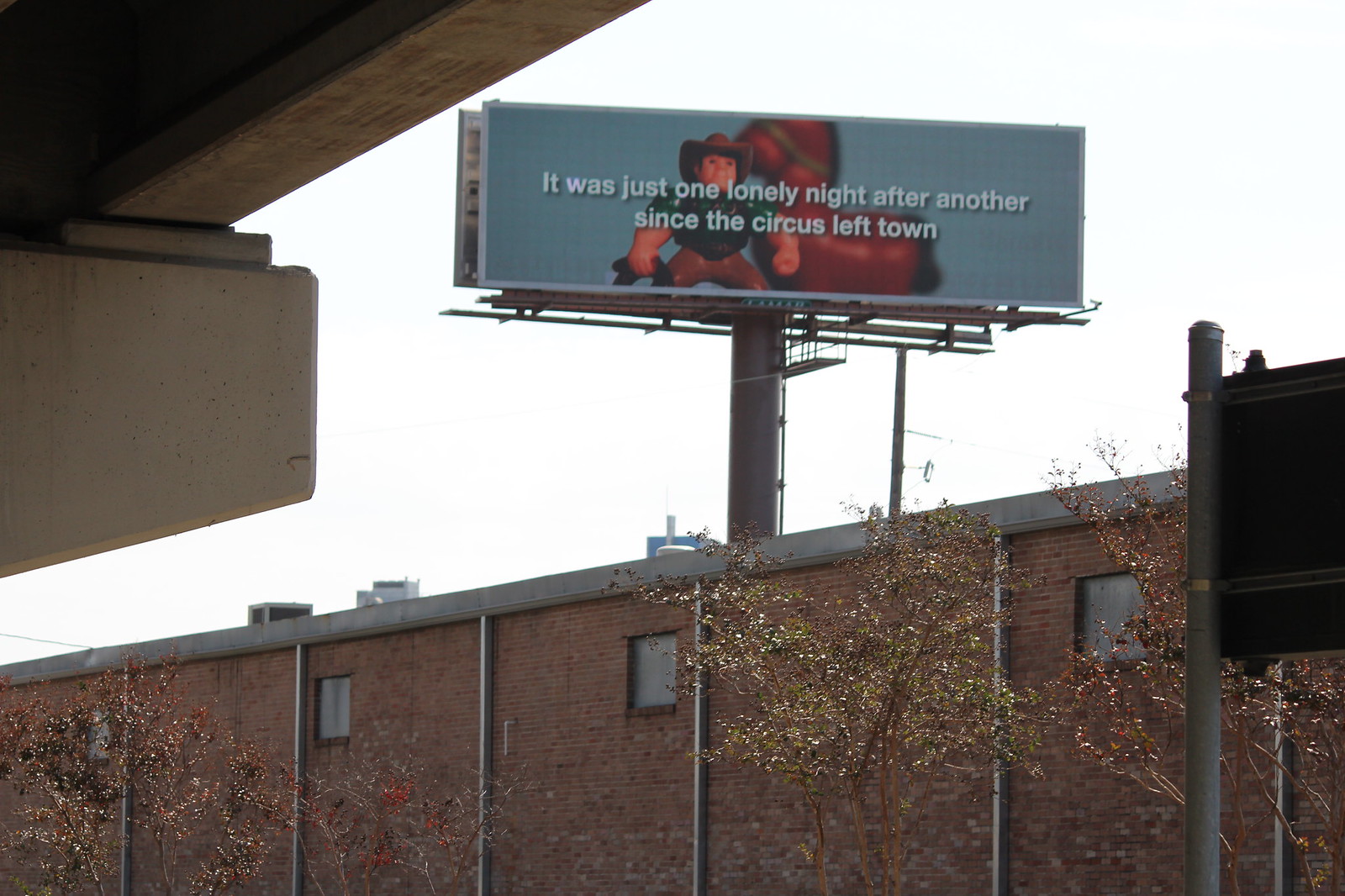This photograph showcases a red brick building with a gray flat roof, adorned with vertical white posts or gutters along its exterior. Its design is minimalist, featuring sparsely placed square gray windows. Occupying the bottom portion of the image, the building contrasts with the upper section, which highlights a wooden rafter and overhang in the top left corner. Centrally positioned atop the building is a billboard depicting a toy cowboy and his toy horse, accompanied by the melancholic words, "It was just one lonely night after another since the circus left town." The sky overhead is a strikingly bright white, providing a stark backdrop. In the foreground, some small trees add a touch of nature, while a traffic sign makes its appearance on the right edge of the lower half of the photograph.